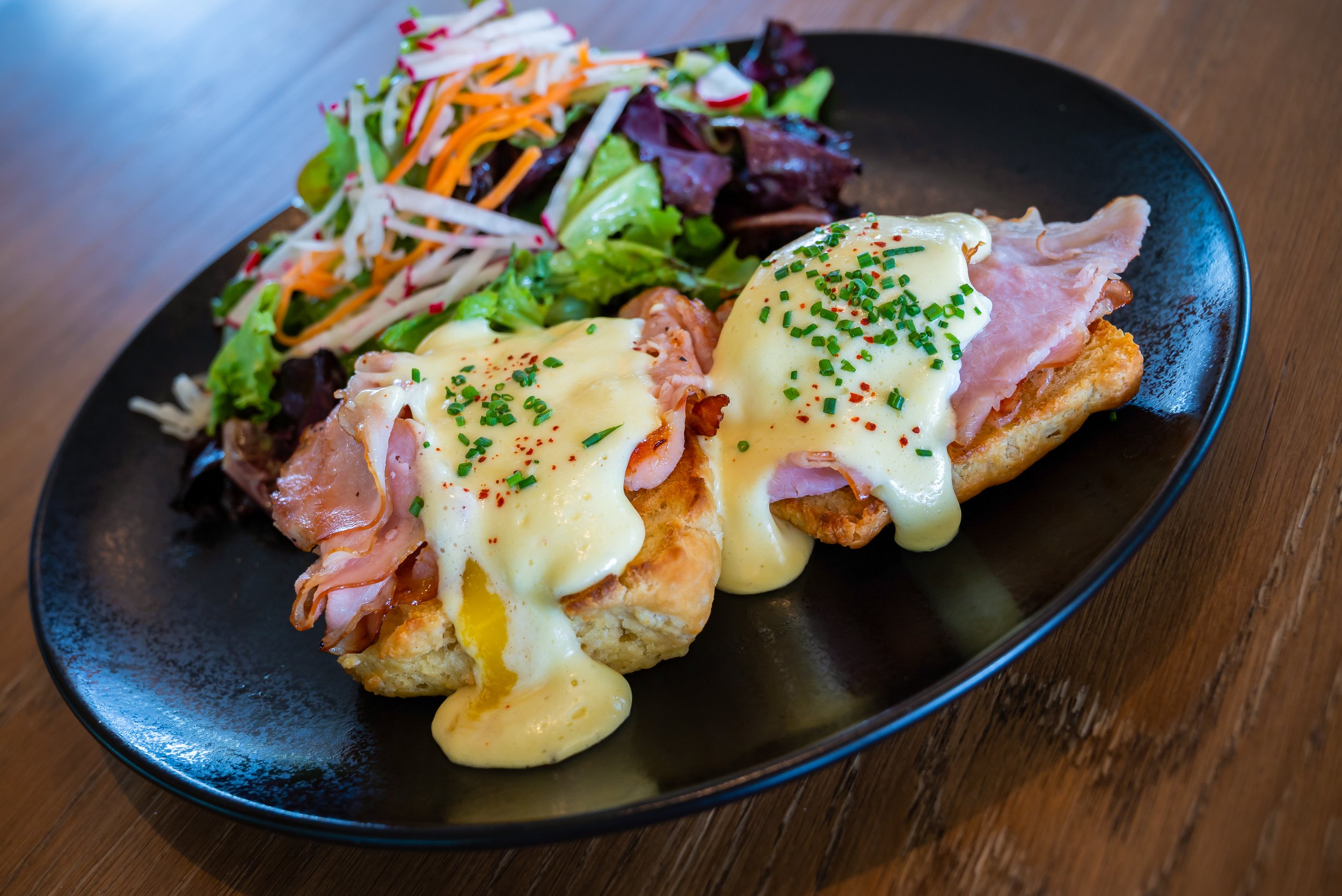This vibrant and mouth-watering Instagram-style close-up image showcases a sophisticated breakfast dish featuring two servings of Eggs Benedict on an elegant, shiny black oval dinner plate. Each serving consists of finely toasted tea cakes, topped with delicious slices of ham, perfectly poached eggs, and luxuriously creamy hollandaise sauce. The eggs are garnished with a sprinkling of vibrant paprika and finely diced chives. Positioned next to the Eggs Benedict is a fresh and colorful side salad, composed of an enticing mix of green and dark red lettuces, grated carrot, and crisp radish slices. The entire setup rests on a dark wooden table, with the photo captured at a slightly off-kilter angle, enhancing the close-up detail and the lush, appetizing appeal of this enticing breakfast scene, seemingly set in an indoor restaurant.